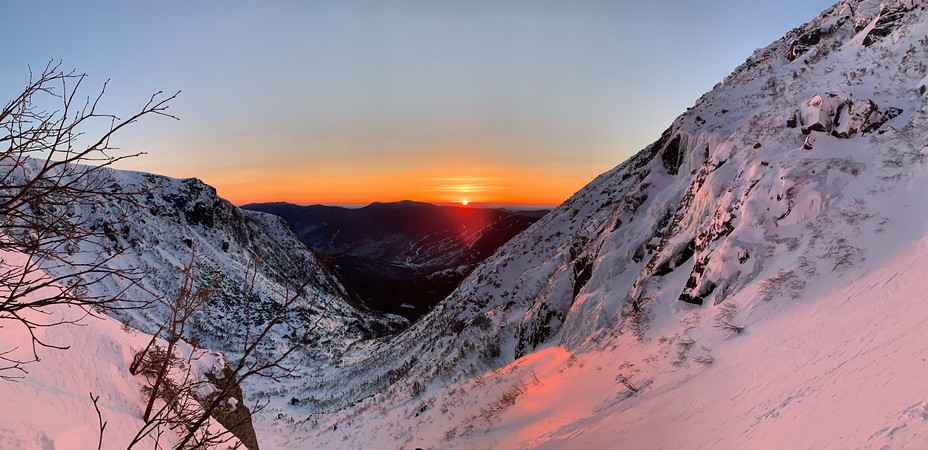This is a wide, horizontally aligned photograph capturing a wintery mountain scene at sunset. The image is taken from a dip in the mountain, with higher elevations visible on the left and right sides, covered predominantly in smooth, white snow. Some brown rock emerges through the snow on the sides of the cliffs, adding texture to the rugged landscape. In the lower left corner, bare branches from a bush or tree protrude, the wiry limbs stark against the white backdrop. The top portion of the photo features a vast, light blue sky with streaks of orange and reddish glow as the sun sets in the distant center, a tiny yellow dot surrounded by soft orange clouds. The V-shaped mountain range descends into a valley, guiding the viewer's gaze towards the glowing horizon where the sunlight gently filters through the scene.